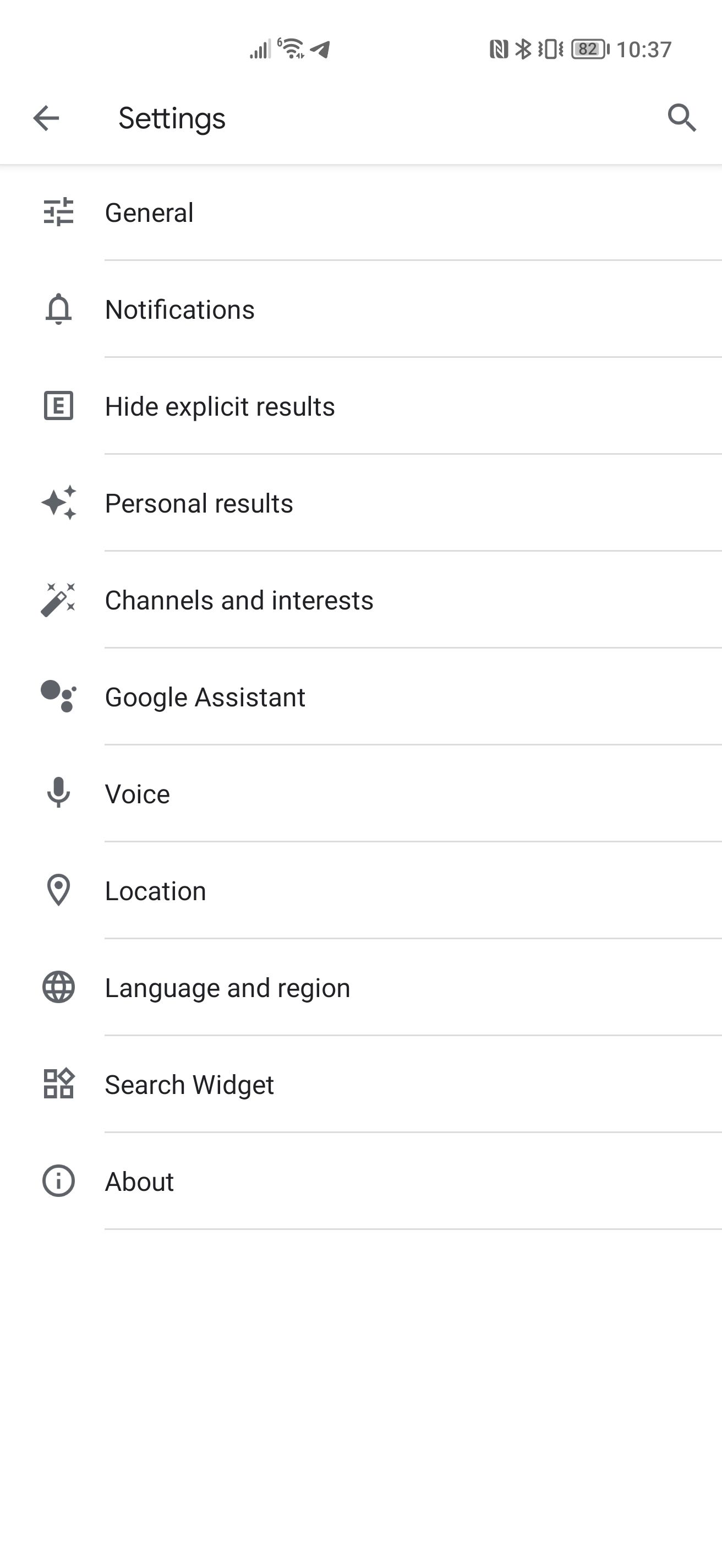This image displays a settings menu on a smartphone with a white background. At the top of the screen, the title "Settings" is prominently displayed with a left-pointing arrow beside it. Below this title, the menu options are listed vertically:

1. **General**
2. **Notifications** – represented by a bell icon.
3. **Hide Explicit Results** – depicted with a small square box containing an "E".
4. **Personal Results** – marked with three stars.
5. **Channels and Interests** – illustrated with a wand icon.
6. **Google Assistant**
7. **Voice**
8. **Location**
9. **Language and Region**
10. **Search Widget**
11. **About**

At the top of the phone screen, various status icons are visible. The signal strength is at four out of five bars, and the Wi-Fi, location, and Bluetooth features are all enabled. The phone appears to be on vibrate mode. The battery level is at 82%, and the current time displayed is 10:37.